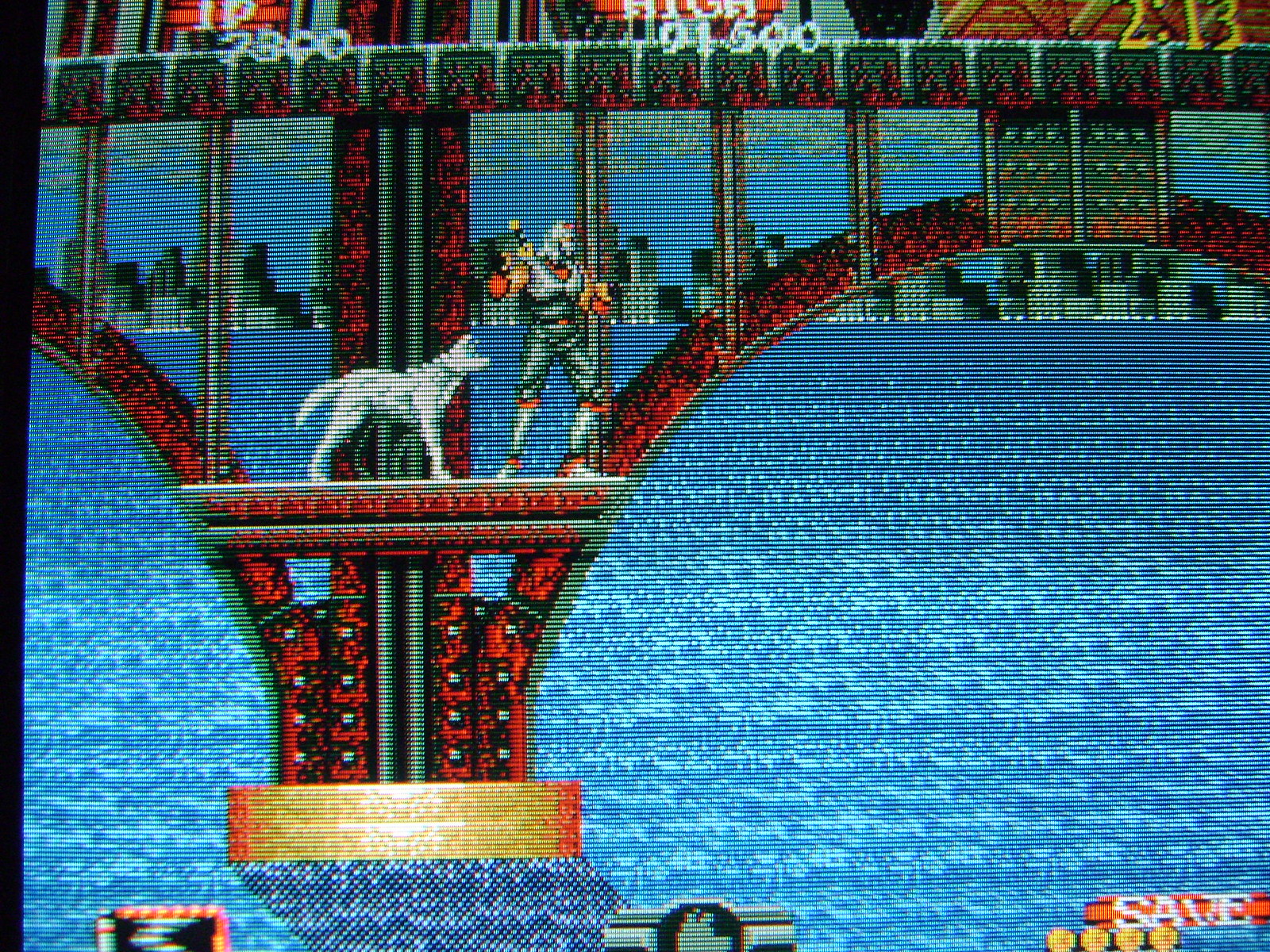This is a detailed screenshot from a straightforward video game. The image prominently features a black and red bridge spanning a river, framed by a distant city skyline. The perspective is up-close, peering through the bridge's structure. Positioned on the bridge, there's a white and grey dog viewed from the side, accompanied by a man in a superhero-esque outfit primarily colored in greys, blues, and light greens. At the top of the screen, a high score of 91,500 is displayed, with the current player's score at 7,300 labeled by "1P." Along the bottom of the screen, there is a "Save" option, indicating game progress can be preserved. The scene captures a quiet moment in the game, set against the backdrop of urban architecture.